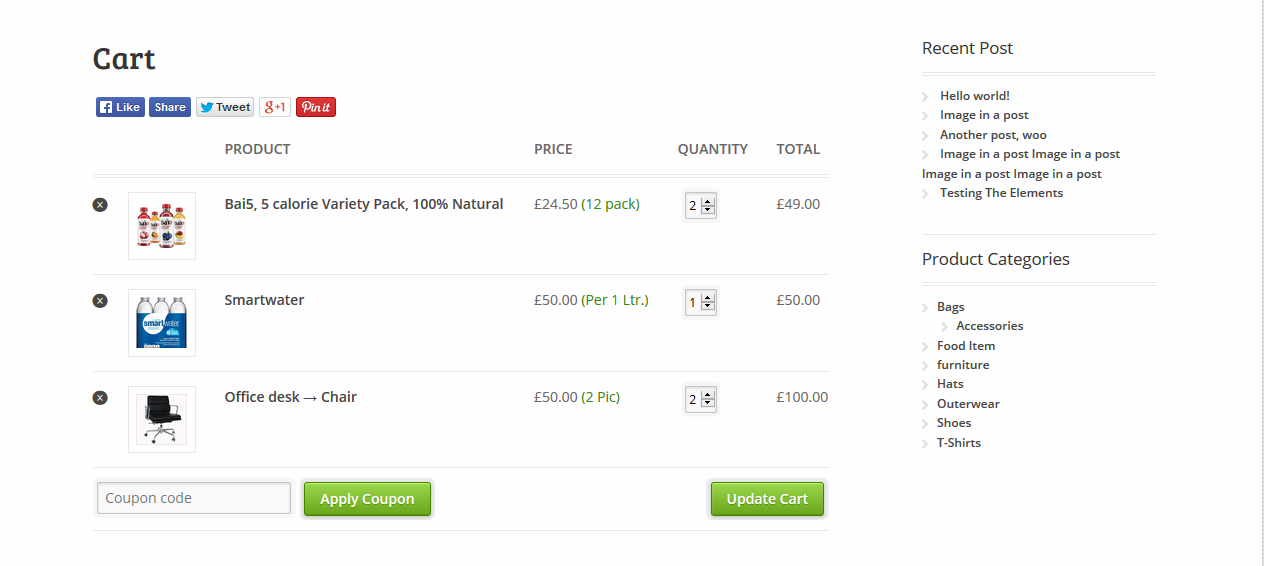The image showcases an online shopping cart on a website with a clean white background. In the upper left corner, the word "Cart" appears prominently in black lettering. Below this, social media links are displayed, allowing users to share their cart on various platforms: "Facebook Like," "Facebook Share," "Tweet," "G+1 for Google," and "Pin it for Pinterest."

Underneath the social media links, the cart's column headers organize the information into categories: "Product," "Price," "Quantity," and "Total." The cart contains three different products, each with its own row. 

To the left of each product line is a black 'X' icon, allowing users to remove items from the cart. Next to the removal icon, images of the products are displayed. Each product entry includes a detailed description: the first product is "Buy Five Variety Pack - 5 Calorie, 100% Natural," the second product is "Smart Water," and the third product is "Office Desk Chair."

The pricing information follows: two packages of the "Buy Five Variety Pack," one unit of "Smart Water," and two "Office Desk Chairs" are listed with their respective prices. 

At the bottom of the cart, there is a section where users can enter a coupon code, along with a clickable link to apply the coupon. To the right, a link labeled "Update Cart" allows users to refresh the cart's contents.